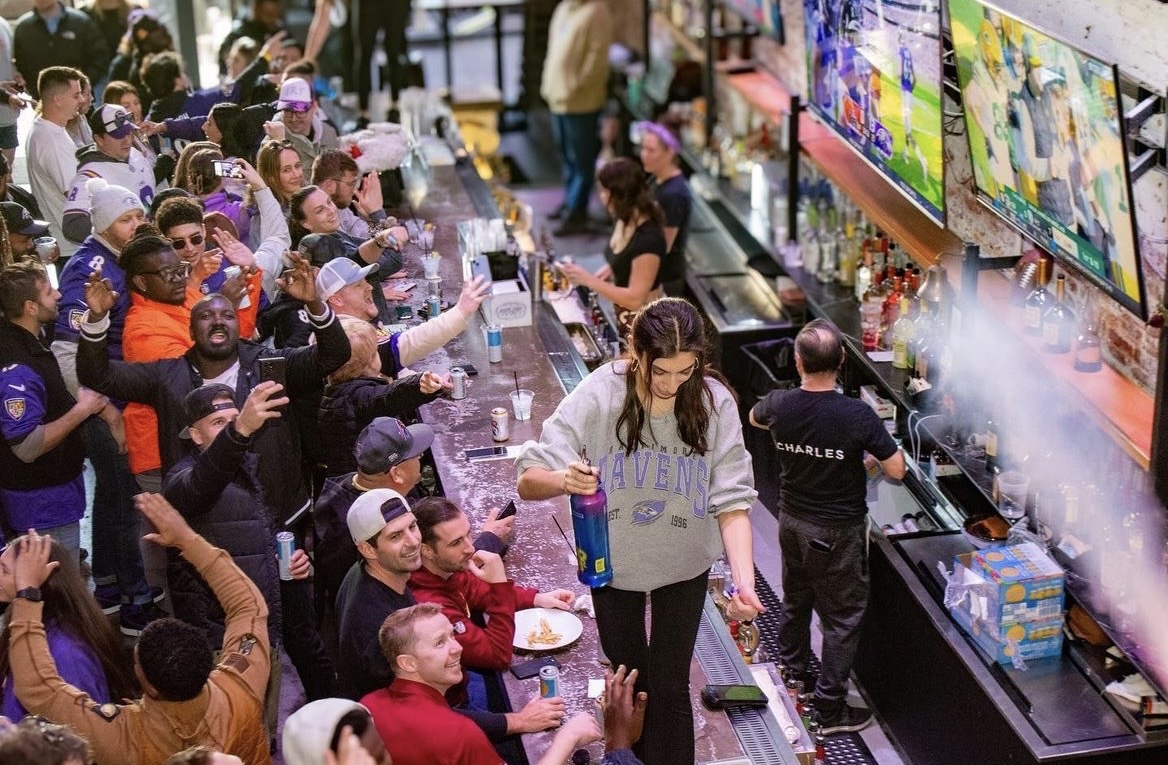The image captures the lively scene inside a bustling sports bar, packed wall-to-wall with enthusiastic patrons. In the very center, a woman donning a grey Ravens sweatshirt and black pants confidently walks atop the cluttered bar, carrying a bottle of alcohol. She has her hair tied back and her gaze directed downward. Behind her, a bartender wearing a black shirt with "Charles" emblazoned on the back attends to tasks alongside two blurred female bartenders. The bar counter is an absolute mess, strewn with cups, plates, and beers. The patron side of the bar is brimming with people, a tapestry of diverse individuals sporting various football jerseys. Notably, one man in the middle of the crowd has his hands raised in the air, seemingly in celebration. Adding to the sports-centric atmosphere, two flat screen TVs in the upper right corner display different football scenes, including what appears to be a Packers game. The crowd's animated expressions and raised hands suggest their team, likely the Ravens, has just made a significant play, filling the bar with palpable excitement and camaraderie.